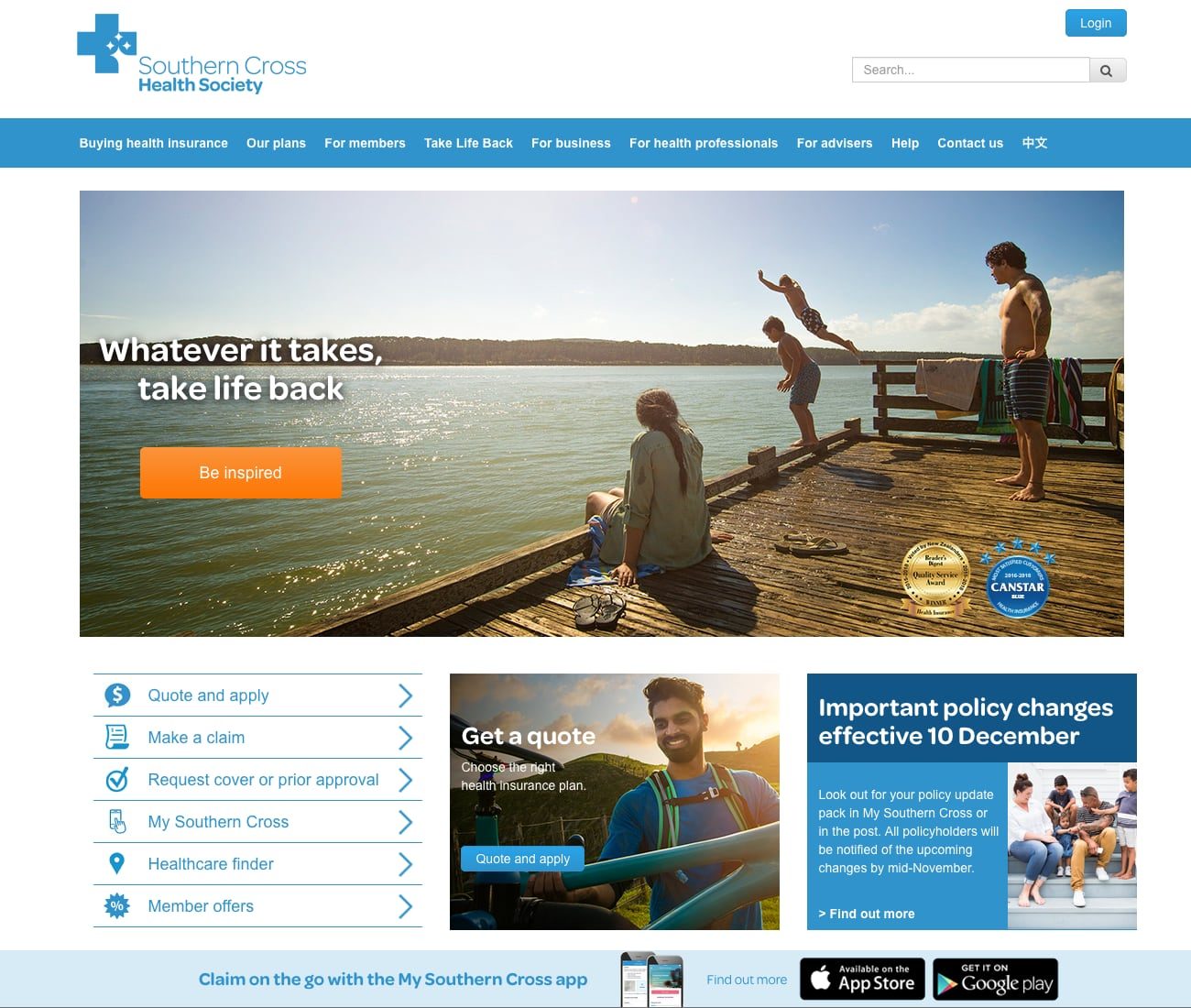The image features a white background with a blue cross in the top left corner, accompanied by the text "Southern Cross Health Society." In the top right corner, there's a blue "Login" button and below it, a search bar. Underneath, a blue rectangular menu appears, albeit slightly zoomed in and blurry, with the following navigational links: "Buying Health Insurance," "Our Plans," "For Members," "Take Life Back," "For Business or Health Professionals," "Advisors," and "Help and Contact Us." Below the menu, there is a serene picture of a lake with calm water, blue skies, and distant trees. A woman is sitting on a pier with her legs dangling over the edge, while two children are diving into the water. Nearby, a man or older teenager in swimming trunks stands watching the children. On the left side of the image are the words "Whatever it takes, take life back," and below that, an orange box with the text "Be inspired."